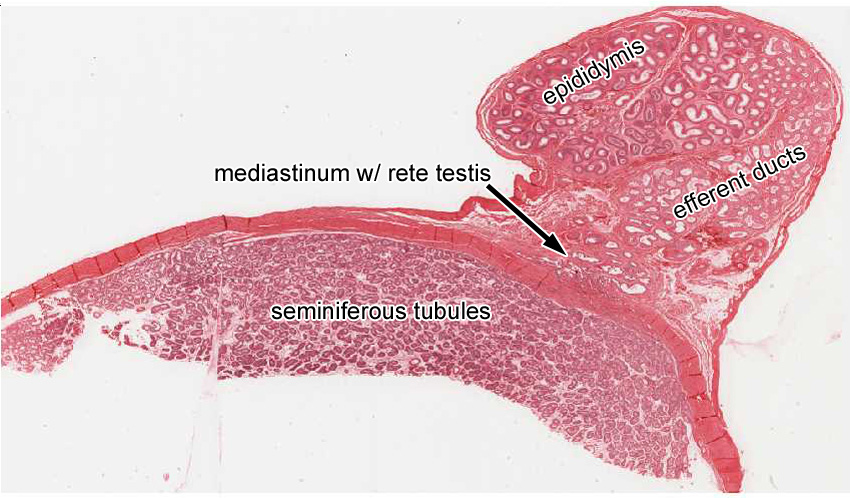The scientific image appears to be a detailed medical illustration on a predominantly white background, showcasing a pinkish-reddish, globular structure with some irregularity to its overall form, likely representing a section of the male reproductive system. Key features labeled within the image include 'mediastinum with rete testis' centrally, 'epididymis' at the top, 'efferent ducts' below it, and 'seminiferous tubules' near the bottom. The detailed annotations are in small black text, suggesting this may be an educational tool used in medical science to illustrate the internal anatomy of a testicle, likely highlighting various functional components such as the seminiferous tubules where sperm production occurs, the efferent ducts which transport sperm, and the mediastinum with rete testis, which are important for sperm maturation and transport. The image could potentially be used for educational purposes, such as teaching about the male reproductive system or associated medical conditions like testicular cancer.